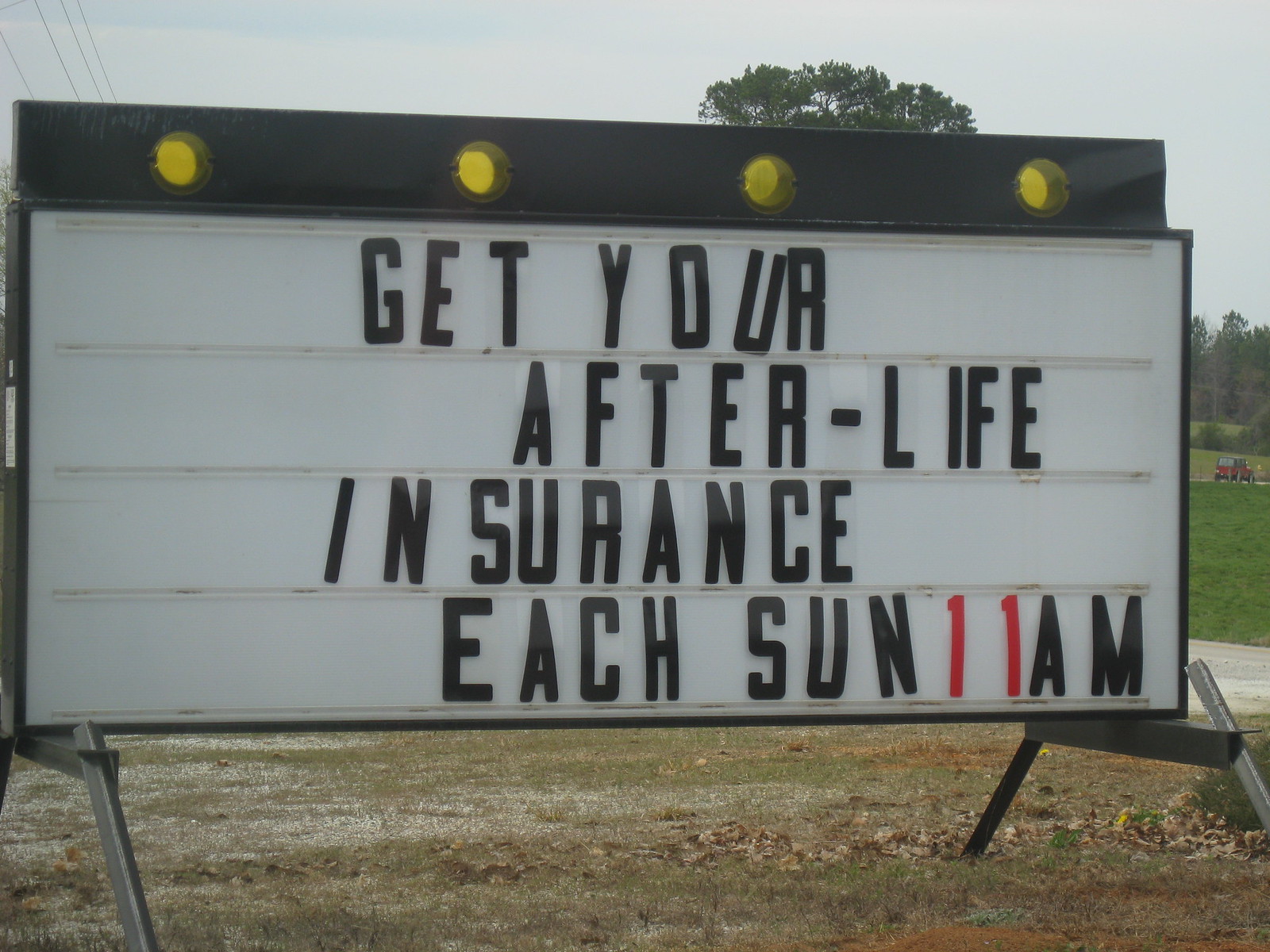This close-up photograph captures a comically styled, weathered sign advertising "Get Your Afterlife Insurance Each Sunday at 11." The humorously intended message is presented with a number of imperfections: the letter "U" is about to fall off, and several letters, particularly the "I" and the "N," are misaligned and spaced unevenly. The sign itself is mounted on two saw horses, the kind typically used in carpentry for cutting wood, adding to its makeshift appearance.

The sign boasts a black trim with noticeable holes along its top border, suggesting age or repeated use. In the background, a large tree and a red tractor are discernible, hinting at a rural or suburban setting. A sidewalk, walkway, or driveway runs nearby, adding to the scene’s detailed authenticity.